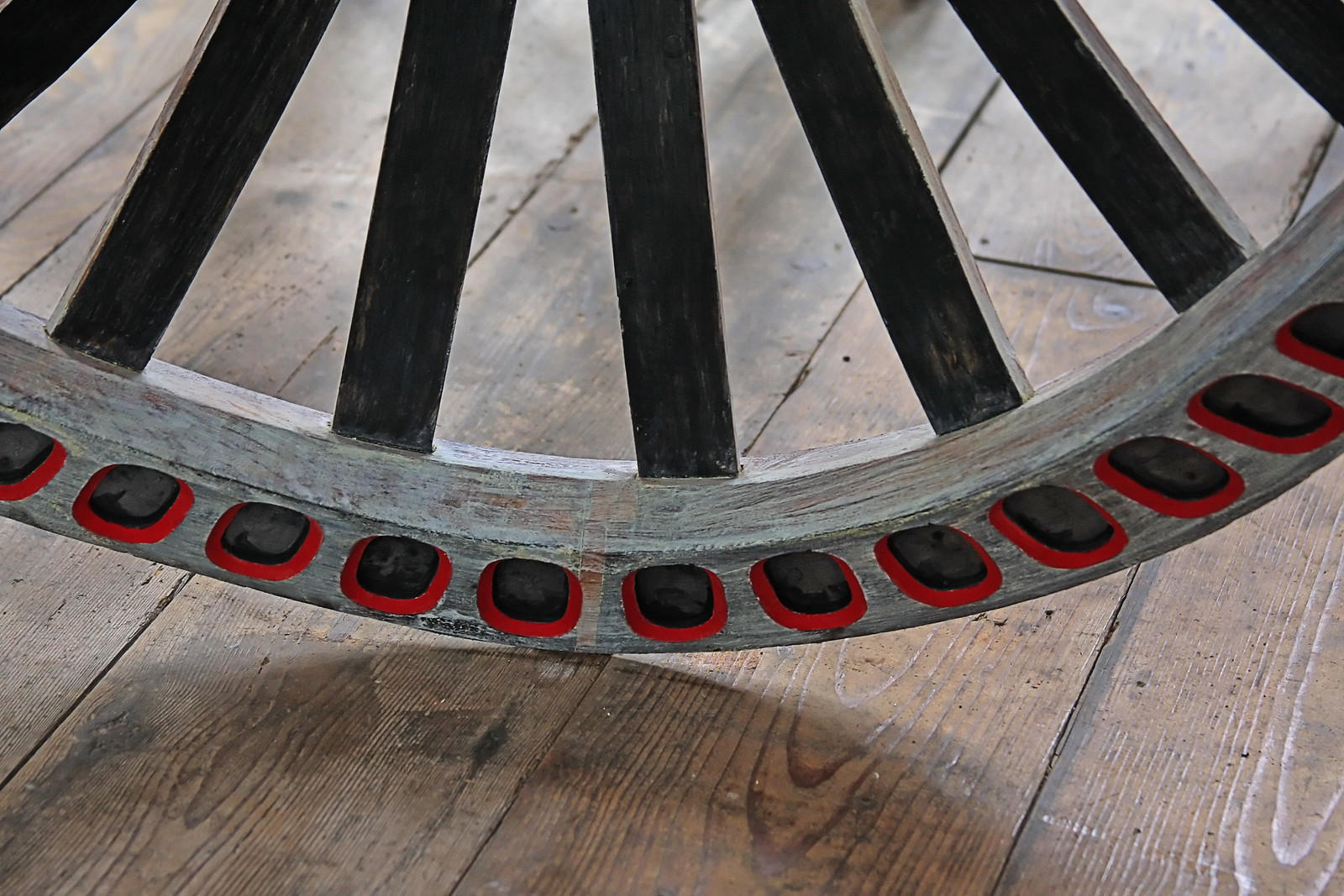This is a detailed landscape-style color photograph depicting a close-up of a wooden wheel resting on a rustic, weathered wooden floor. The floor consists of brown planks with visible grain and signs of wear, enhancing its rugged, aged appearance. The wheel, which is predominantly gray, features several flat, dark gray spokes that extend from its inner rim towards its unseen center. The visible portion of the wheel shows seven wooden spokes arranged at a slight slant. Encircling the outer edge of the wheel are approximately twelve oval-shaped indentations with rounded corners. These indentations are bordered in red with black centers, adding a distinct contrast to the muted gray of the wood. The image is artistically cropped, focusing on a segment of the wheel, leaving its complete structure and surroundings to the viewer's imagination.